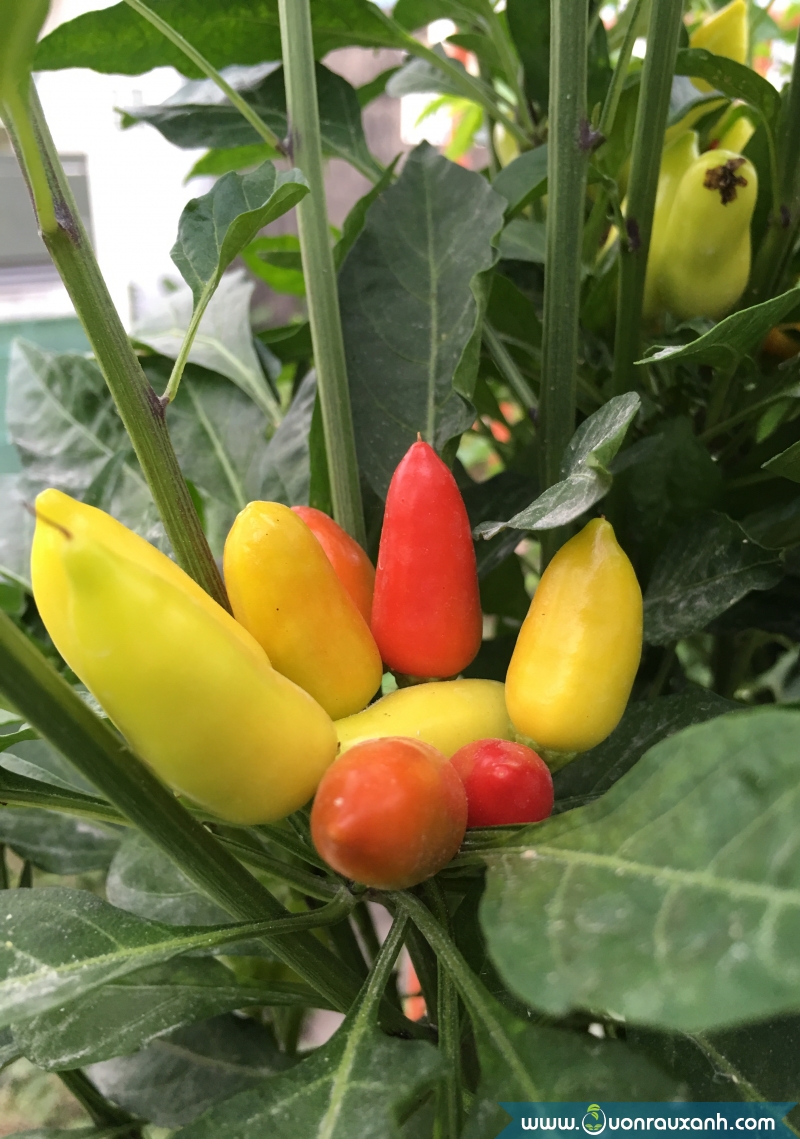This detailed image captures a close-up of a vibrant outdoor garden scene featuring a cluster of tubular vegetables, most likely a variety of banana peppers. The focal point of the photo is a dense pile of these peppers growing from a central stalk adorned with lush green leaves and long stems. The peppers display a vivid spectrum of colors, transitioning from yellow to red, indicating different stages of ripeness. Yellow peppers dominate the center, with some red ones interspersed among them. Additional leaves and ripe peppers populate the background, alongside a muted white wall visible towards the left side of the frame, suggesting an outdoor setting. The bottom of the image features a website URL, "www.uonrauxanh.com," in white letters within a green box. Overall, the photo is teeming with the natural growth and richness of this pepper plant, set against a backdrop of greenery and distant architecture.